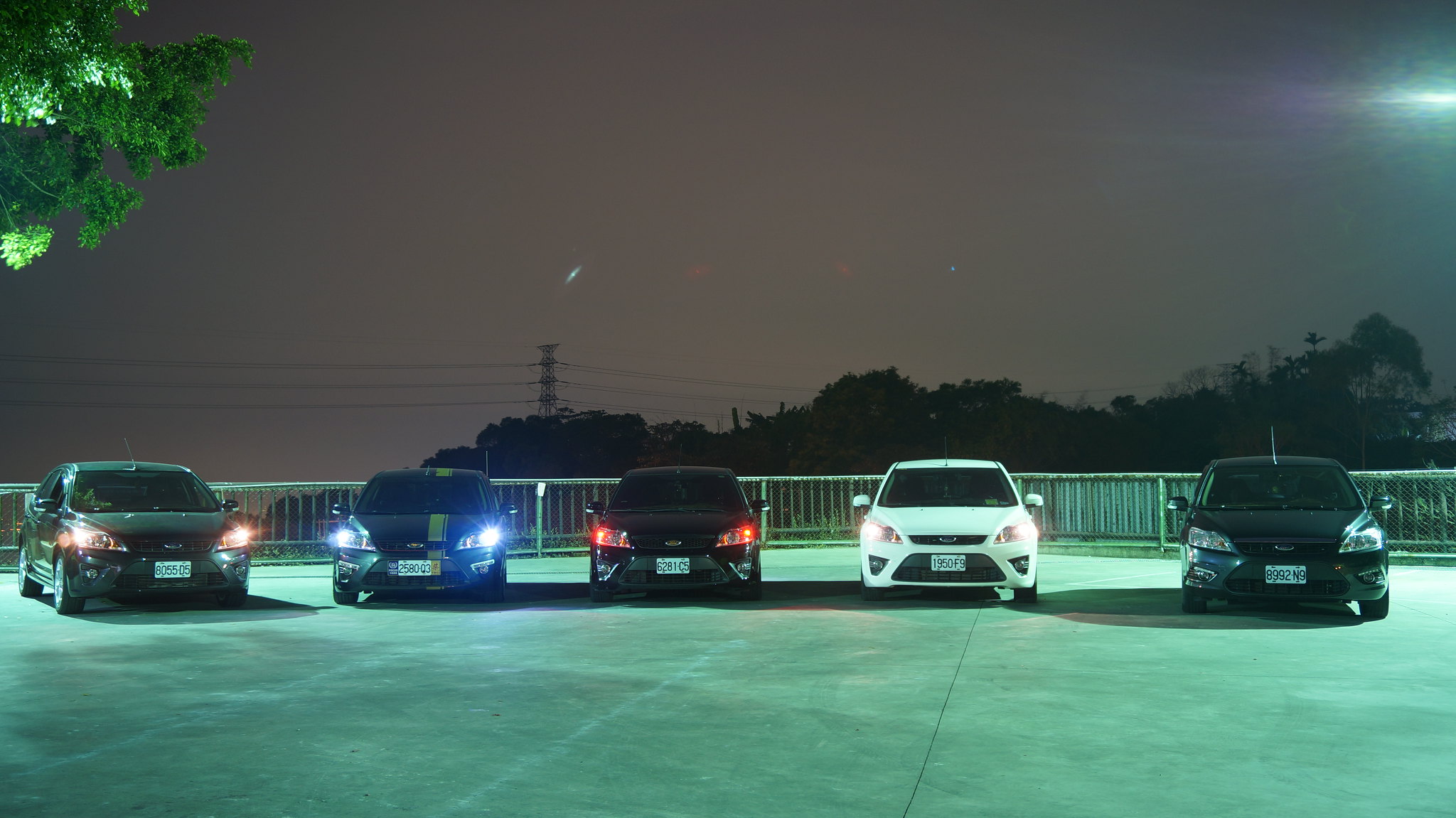The image captures a nighttime scene of an elevated parking lot with a cement ground surface. The parking lot is demarcated by a metal fence in the background. The sky exhibits a dark brownish-gray hue, possibly indicating the period just after sunset or before sunrise, with a slight pink tint. The lighting conditions are low, rendering the scene quite dark. 

In the foreground, five cars are lined up facing the viewer. Starting from left to right, the first car appears gray, followed by a black car with a vertical white stripe down its entire body, another black car, a white car, and a final dark-colored car, possibly black or gray. Notably, the first four cars have their headlights on, while the car on the far right does not.

In the upper left corner of the image, there is tree foliage visible. The top center features a tower-like structure in the distance, and a light source illuminates the upper right corner, contributing to the overall moody ambiance of this nighttime parking scene.